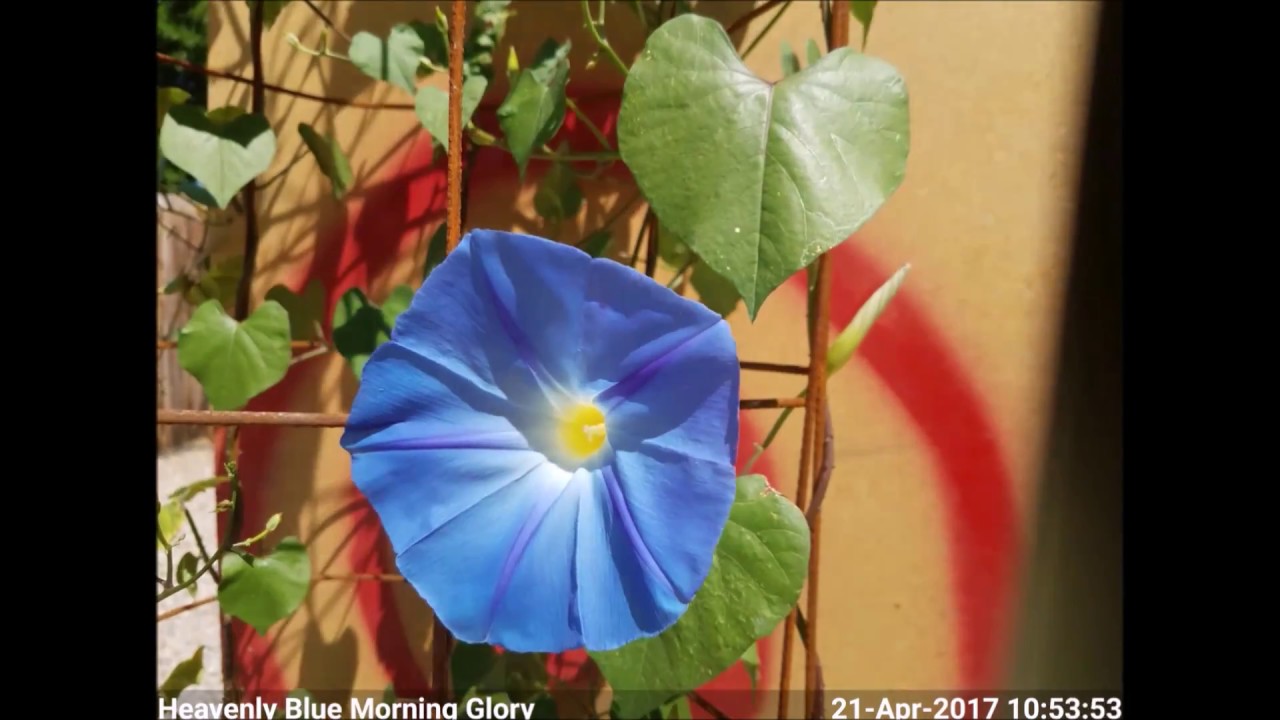A close-up photograph features a large blue flower with a yellow center, identified as a "Heavenly Blue Morning Glory." The petals are blue with a hint of purple in between, and they appear to be fused together. The flower is situated amidst several green vines and leaves that are winding around a man-made object with a grid pattern. The background of the image is slightly out of focus but seems to depict a tan wall with red circular markings, possibly resembling a target. Both the left and right sides of the image are bordered by black vertical bars. At the bottom left corner, the text reads "Heavenly Blue Morning Glory" in white, and on the bottom right corner, the date and time "21-APR-2017, 10:53:53" are displayed in white text. The predominant colors in the image include blue, yellow, green, red, tan, black, and white.